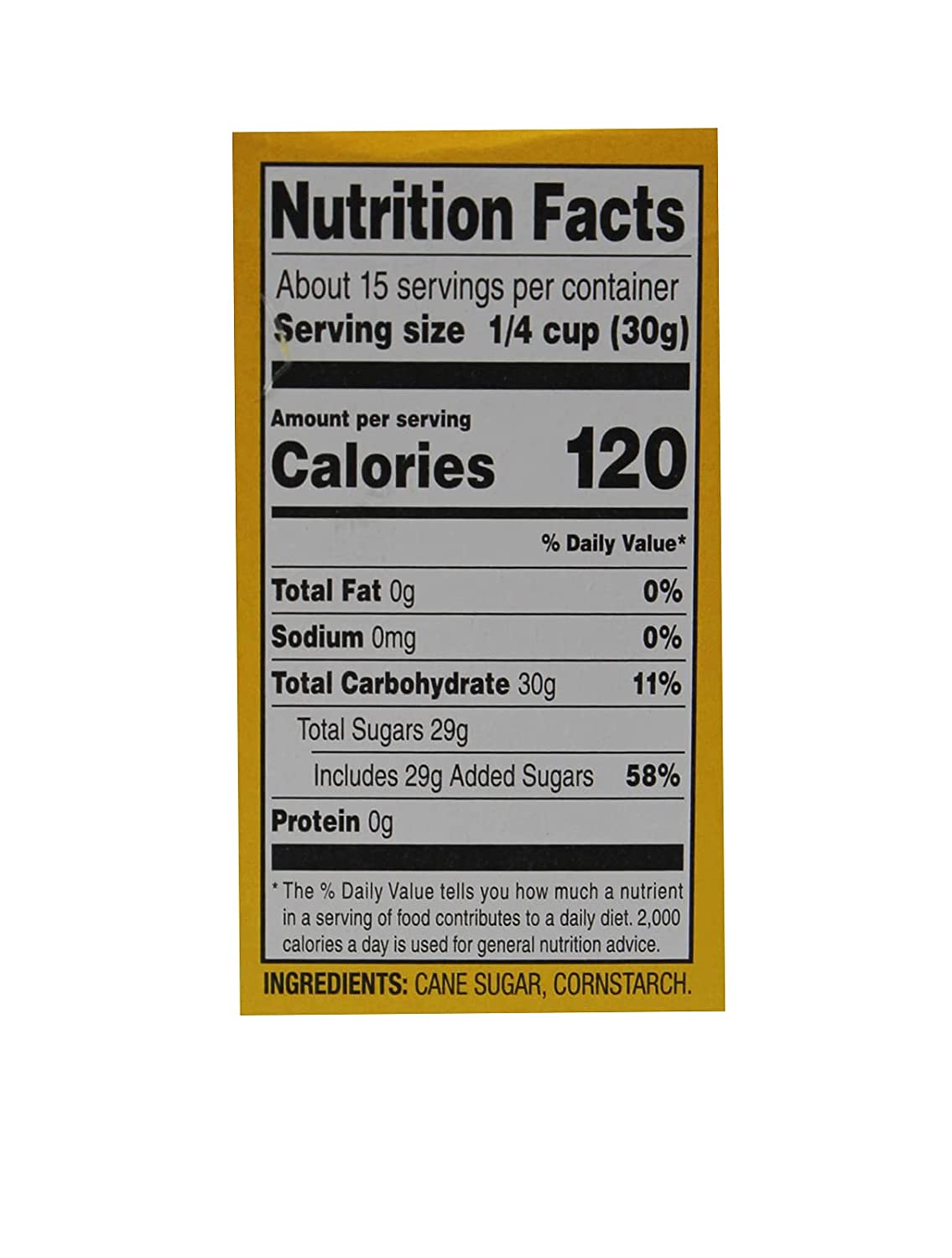This image showcases a comprehensive Nutrition Facts label on a white background with black lines demarcating different sections. It details that there are about 15 servings per container, with a serving size of a quarter cup (30 grams). Each serving provides 120 calories. Key nutritional information includes 0 grams of total fat, 0 milligrams of sodium, 30 grams of total carbohydrates (which equates to 11% of the daily value), 29 grams of total sugars including 29 grams of added sugars (accounting for 58% of the daily value), and 0 grams of protein. The label emphasizes that this information helps determine how much a nutrient in a serving of food contributes to a daily diet based on a 2,000-calorie intake. The ingredients listed are cane sugar and cornstarch, which suggests the product might be powdered sugar. The label takes up most of the image, with the overall background appearing yellow.